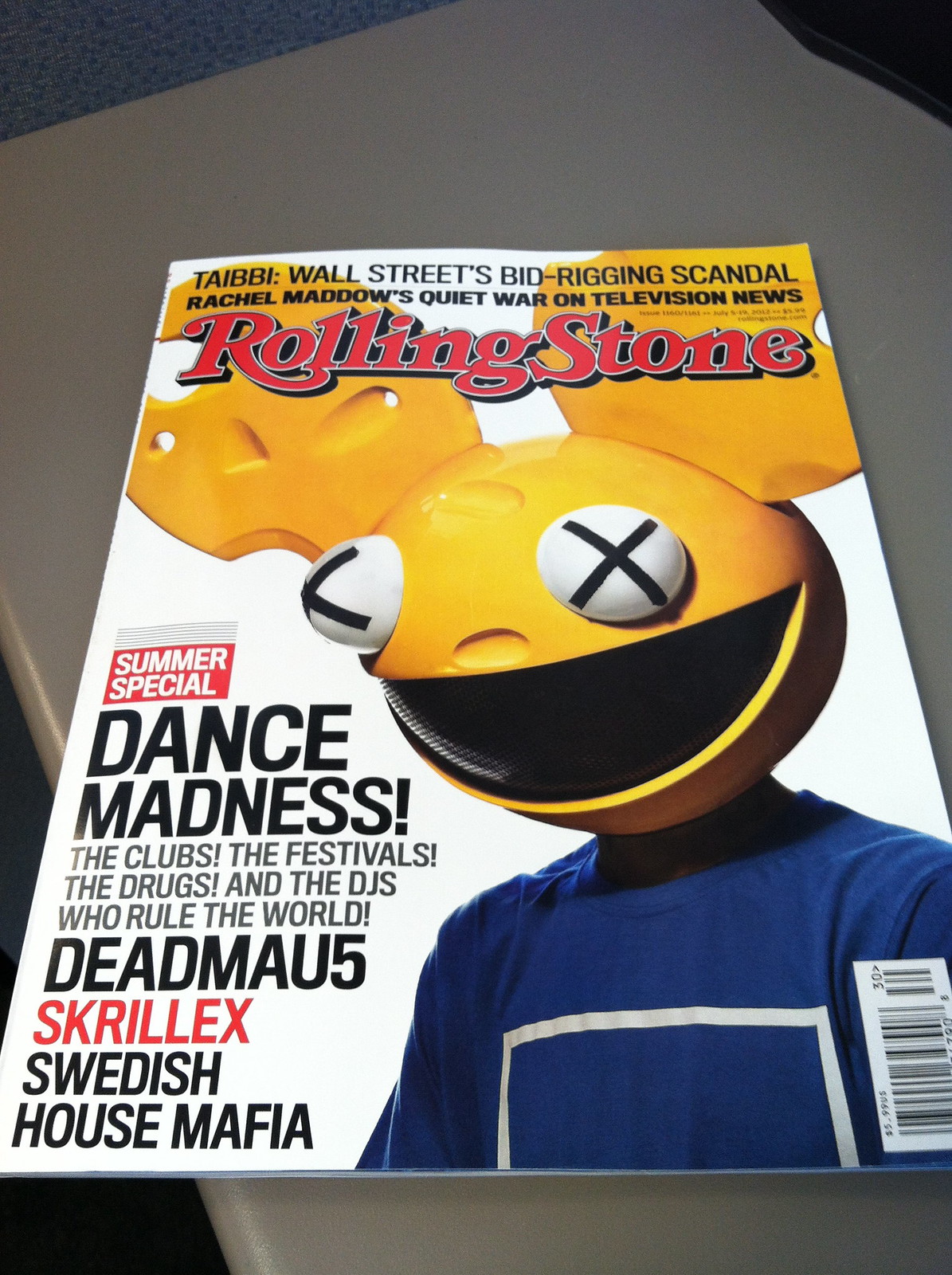This detailed caption combines and highlights the common elements from the three inputs:

This image shows a copy of Rolling Stone magazine placed flat on a gray, possibly white, surface. The magazine cover prominently features the iconic red Rolling Stone logo at the top, set against a predominantly white background. Above the logo are a few lines of black text. Dominating the center-left section of the cover is a cartoonish, animated figure resembling Deadmau5, characterized by a yellow head with large, moose-like ears. The head features white, round eyes with black X's over them, and a wide-open black mouth. This figure is wearing a blue shirt with white lines that form a rectangular outline across the chest. Positioned along the left side of the cover, in bold text, are the words “Summer Special” in red, followed by "Dance Madness" in large black letters with an exclamation point. Below this, there are three lines of less bold black writing about clubs, festivals, drugs, and DJs, listing notable names like Deadmau5, Skrillex, and Swedish House Mafia. A barcode appears in the bottom right corner, partially overlapping the left arm of the figure.